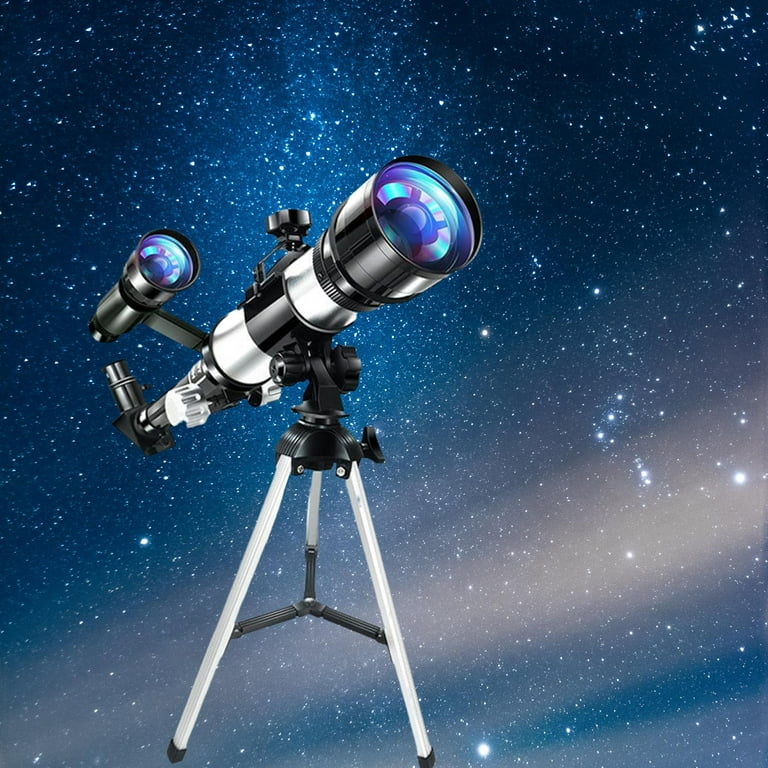The image is a detailed and vibrant depiction of a telescope set against a dark blue night sky teeming with thousands of stars. These stars, appearing as tiny white and turquoise specks, dot the entire background, evoking a cosmic, spacey ambiance. The night sky also features subtle, lighter rays of light that pierce through the darkness at the bottom of the image, adding depth and dimension.

The telescope itself is mounted on three silver legs, structured in a tripod formation for stability, with black covers on the foot ends and additional black connecting bars. The main body of the telescope is black and features two prominent lenses: a larger, slightly purple-tinged lens at the front and a smaller lens mounted towards the back. These lenses give off reflections of both purple and light blue hues. A black plastic eyepiece is situated at the end, and a knob atop the telescope allows the viewer to adjust the focus. This intricate and captivating product image effectively merges the majestic, star-filled night sky with the functional elegance of a high-quality telescope.